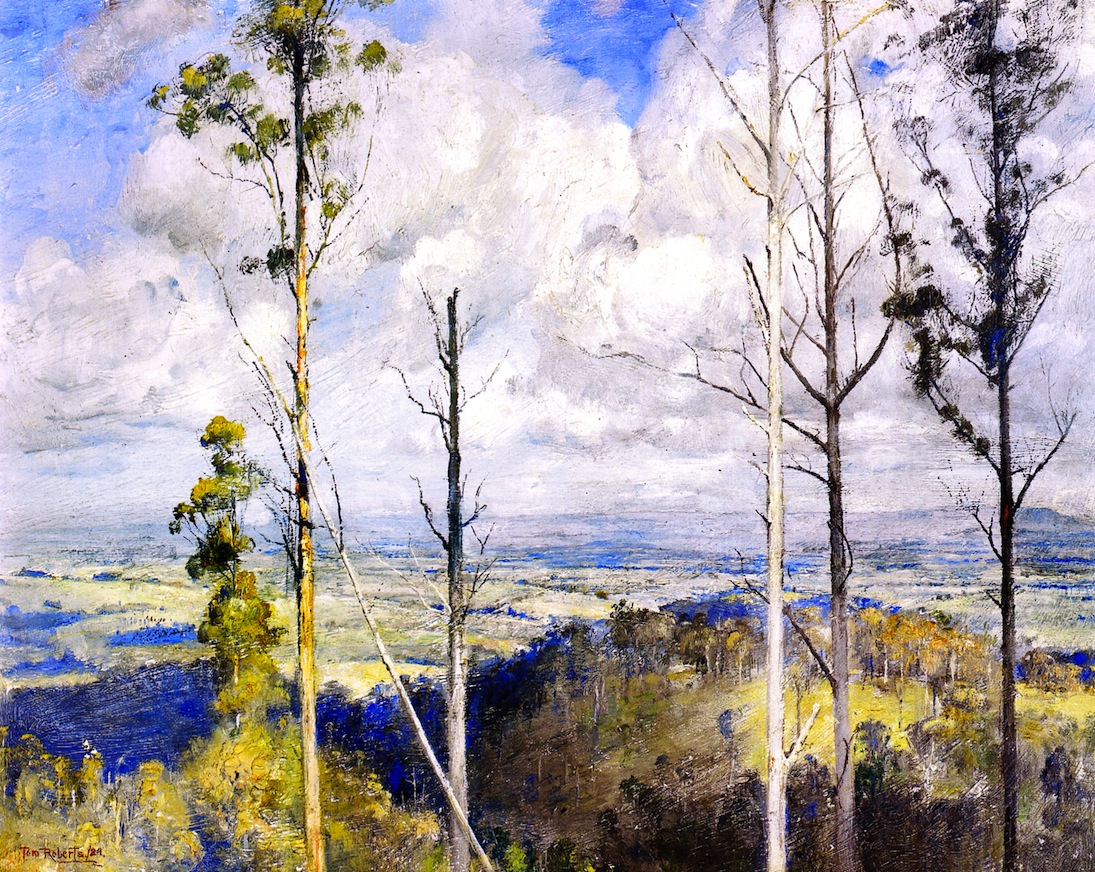The image depicts an abstract painting of a landscape captured from an elevated perspective, possibly from the top of a hill or mountain. The scene features a mix of bare, thin, white tree trunks interspersed with a few scattered evergreen trees, creating a striking contrast. The foreground includes multiple tree trunks, with three on the right side and two on the left; among these, a particularly thin tree leans diagonally against the others on the left. The trees are largely leafless, adding to the stark and serene atmosphere of the scene.

The terrain in the foreground appears to be covered in yellow-green brushstrokes, suggesting grassy or brushy land. There are also hints of darker green patches, some described as slightly hilly, adding depth to the composition. The middle ground consists of more tree lines and a green patch on a slight hill surrounded by yellow-leaved trees.

In the distance, a flatland extends, possibly indicating a vast stretch of landscape that contrasts with the hilly foreground. Above this scene, the expansive sky is filled predominantly with clouds, though patches of blue are visible, providing a dramatic backdrop to the serene but intricately detailed natural setting.